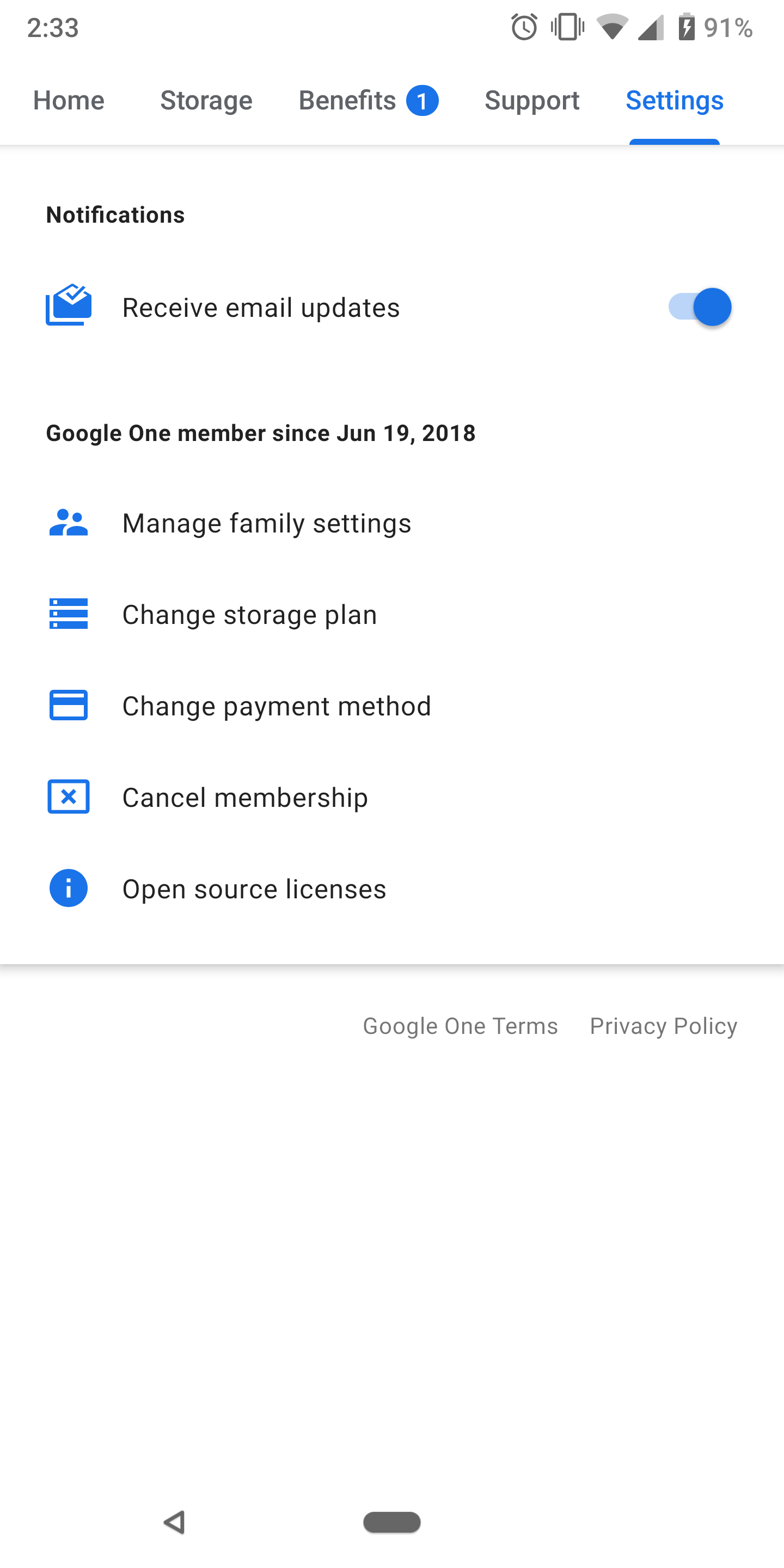Screenshot of a Google One subscription settings screen with a predominantly white background and minimal blue accents. The status bar at the top displays the time as 2:33 PM, with icons indicating an active alarm, vibrate mode, Wi-Fi connection, strong signal strength, and a battery level of 91%. Below the status bar is a navigation menu featuring "Home," "Storage," "Benefits" (labelled with a notification badge showing the number 1), and "Settings," which is highlighted in blue with an underline.

The main content section starts with "Notifications," followed by a mail icon and the option "Receive mail updates," enabled by a blue slider. Further down, text confirms "Google One member since June 19, 2018."

A list of options follows, each accompanied by icons:
- "Manage family settings" with a man and woman icon,
- "Change storage plan" with three stacked rectangles,
- "Change payment method" with a blue wallet icon,
- "Cancel membership" with an X inside a box,
- "Open source licenses" with a lowercase 'i' inside a circle.

At the bottom right, hyperlinks for "Google One terms" and "Privacy policy" are visible.